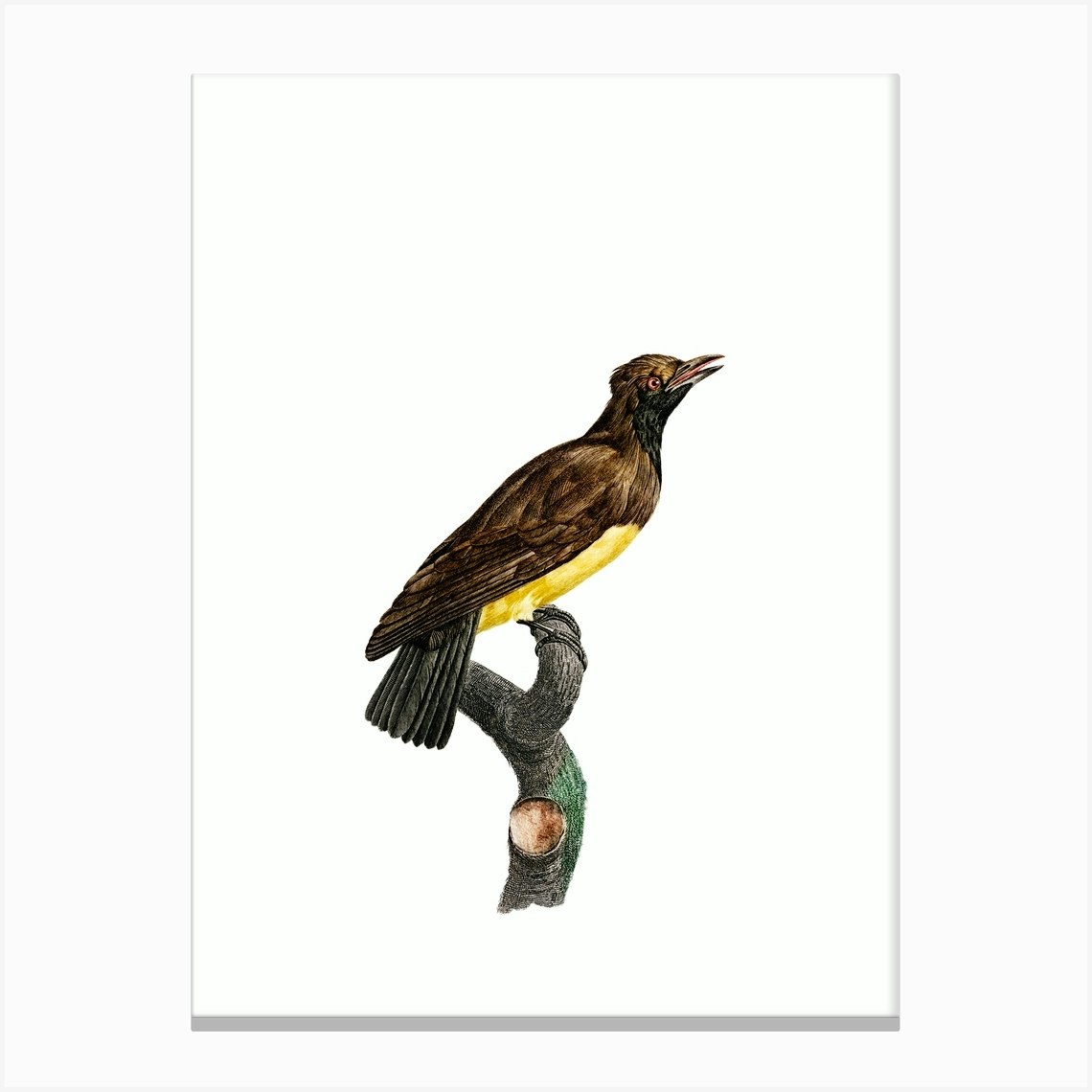The painting depicts a brown bird perched on a tree branch against a white background. The bird faces to the right, showcasing its distinctive coloration: brown on the head and body, a yellow belly, and a black-tipped beak, which is slightly open revealing its tongue. Its red eye is prominently visible, and its black-rimmed tail feathers appear ruffled. The branch, which is substantial but truncated, features a freshly cut knot displaying a pinkish-apricot inner wood and a green paint mark on its side. The bird's claws firmly grasp the branch, and there is a subtle shadow cast at the bottom of the image.